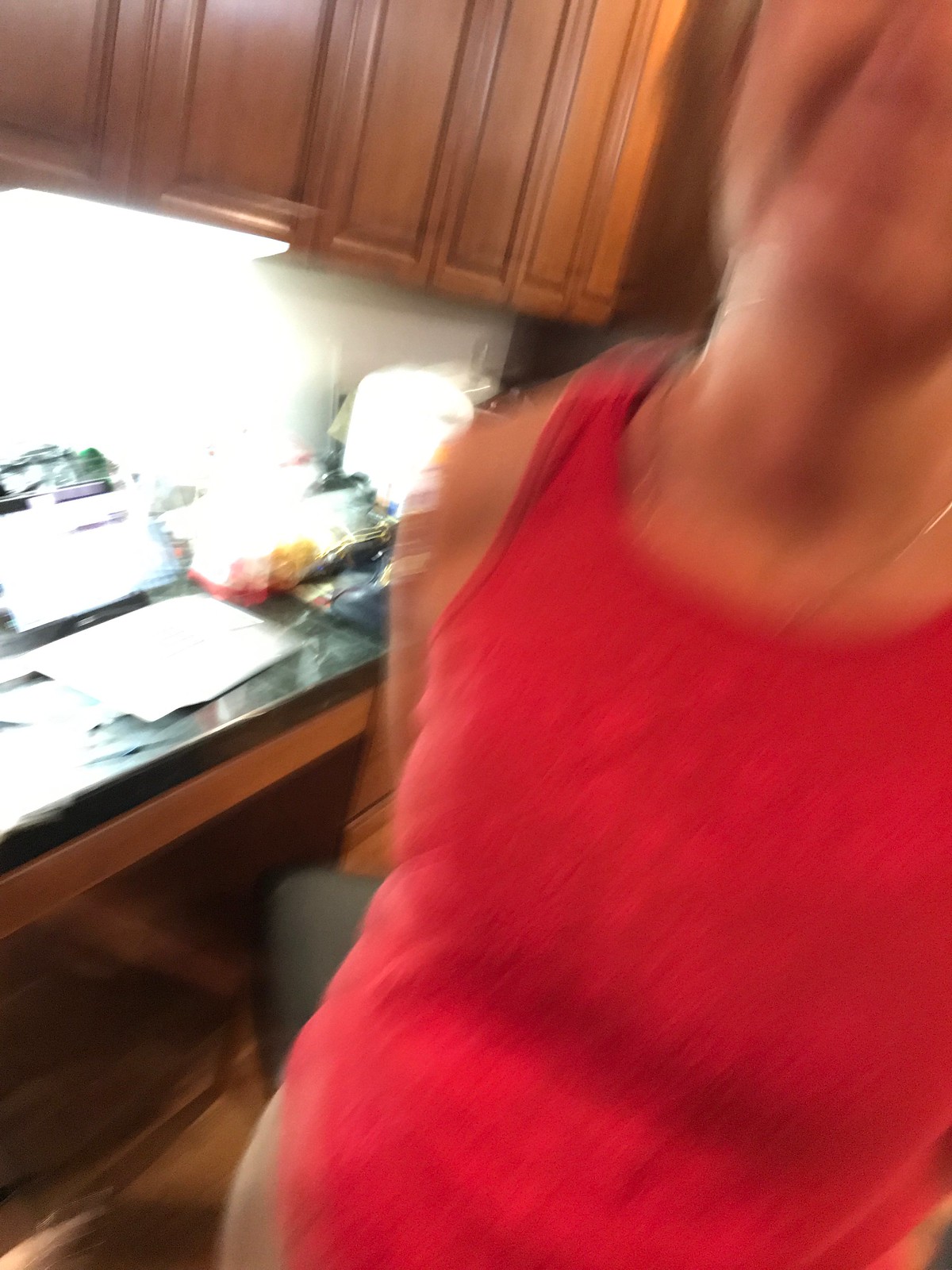The image captures a woman who is slightly out of focus, making the overall photograph a bit blurry. She is partially visible, from the lower part of her face down to about her waist. She is dressed in a red shirt and wears a necklace, paired with what appear to be beige pants, though the clarity is poor. 

In the background, to the left of the woman, there is a black tabletop cluttered with papers and a few indiscernible items, possibly including a lamp and something yellow and red. Above this area, brown cabinets with an under-cabinet white light are visible, casting a bright glare that overexposes part of the scene. 

On the floor, there's a black chair and a piece of carpet adding to the room's texture and depth, even though the overall sharpness of the image is compromised.